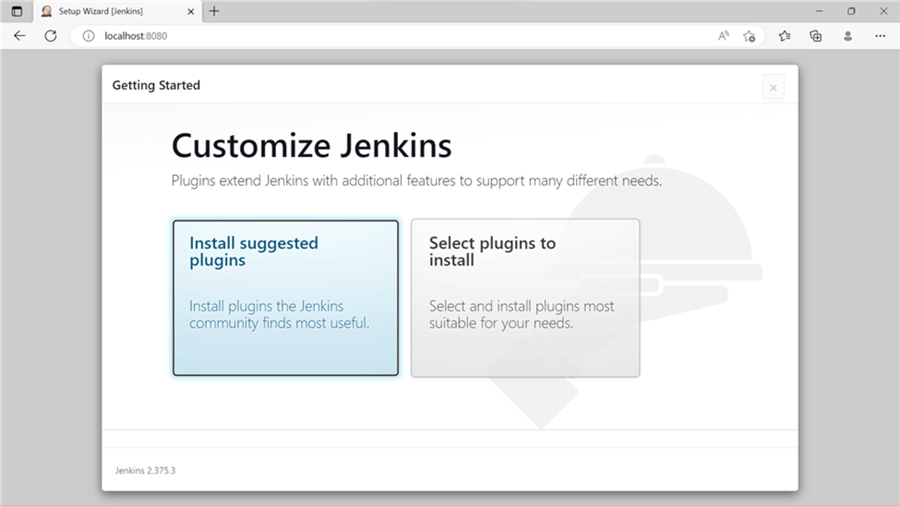Screenshot of the Jenkins Setup Wizard in a web browser:

- **Browser Tab:** One tab labeled "Setup Wizard Jenkins" with a small person icon.
- **Address Bar:** Displays "localhost:8080."
- **Page Content:**
  - **Header:** "Getting Started"
  - **Subheader:** "Customize Jenkins - Plugins extend Jenkins with additional features to support many different needs."
  - **Option Boxes:**
    - **Left Box:**
      - **Background:** Blue
      - **Text:** "Install Suggested Plugins - Install plugins the Jenkins community finds most useful."
    - **Right Box:**
      - **Background:** Light gray
      - **Text:** "Select Plugins to Install - Select and install plugins most suitable for your needs."

Overall, it describes the initial setup steps for Jenkins, highlighting plugin installation options.